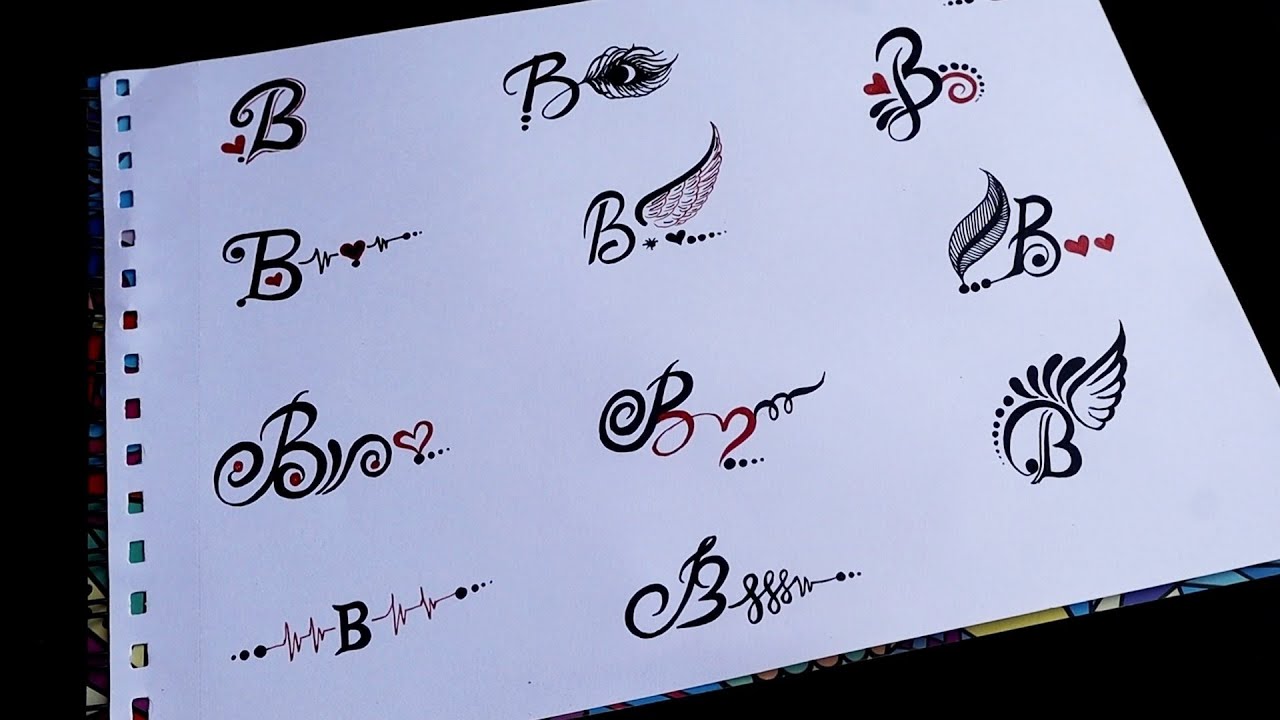This image depicts a piece of white notebook paper with regular perforations along the left-hand side for easy insertion into a scrapbook or album. Set against a black background, the paper showcases 11 distinct and intricately designed styles of the letter "B," rendered in various calligraphy, print, and scripted styles, and presented in black ink. Some designs feature red adornments, particularly hearts.

In the top left corner, there's a B with a small heart behind it. Just to the right, another B features a peacock feather extending from below. On the next row, the first B includes a heart in the bottom loop, followed by a B decorated with an echocardiogram symbol and a heart in its center. Next to this, a B is embellished with an angel wing extending to the right, accompanied by a heart and several trailing dots. To its right, you'll find a B with a flourish and dots emanating from the side, also featuring a heart.

On the row below are even more inventive designs. The first B on this line is highly ornate, adorned with multiple loops, a heart, and trailing dots. To the right is a B with a curved tail, where the second loop forms the arches of a heart with two small swirls extending from it. Further right, a B is integrated with a feather that leads from dots, culminating in several hearts in front of it.

In the bottom left, there is a B intersected by echocardiogram spikes, indicating a heartbeat, with the letter positioned centrally. To its immediate right, a B is decorated with several graceful, S-shaped swirls transforming into dots. Finally, the bottom right-hand corner features a B with dots along the top arch, culminating in an angel wing outline.

The page could serve various decorative purposes, such as insignias on stationery, monograms, or even tattoo designs.